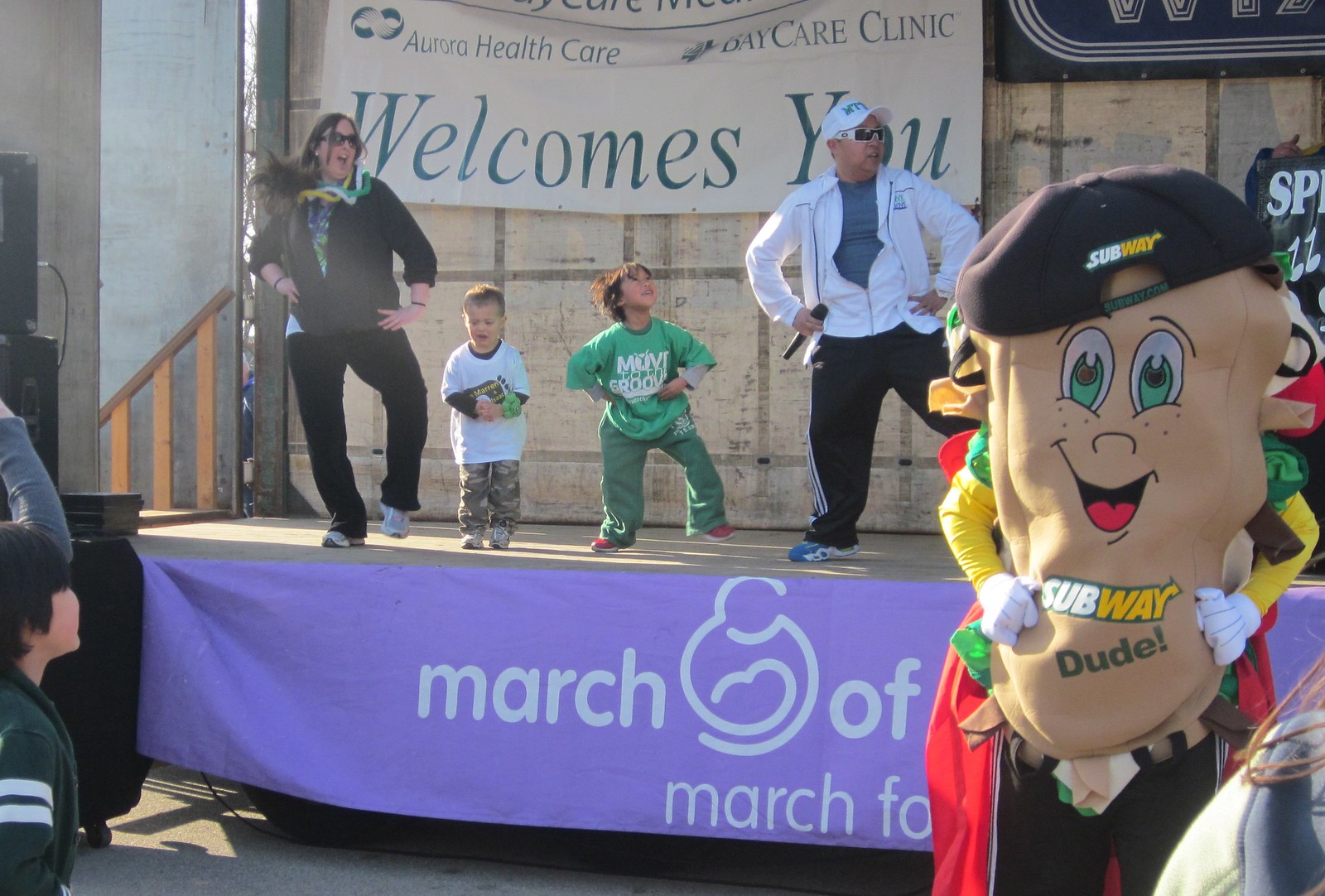This vibrant color photograph captures an outdoor stage performance featuring an adult woman, an adult man, and several children dancing. Central to the image is a lively scene with dancers arranged from left to right: a smiling woman in sunglasses, a fleece zip-up jacket, dark pants, and adorned with green, white, and yellow plastic leis. Next to her, a young child in camouflage pants and a white t-shirt is crying, while another child, dressed entirely in green, dances energetically with his hands on his hips. To their right, a man wearing a white baseball cap, a white zip-up jacket over a blue shirt, and black pants is also dancing with his hands on his hips, holding a microphone in his right hand. The stage decor includes a prominent blue banner that reads "March of Dimes" and features the organization's logo. A larger white banner in the background, adorned with green text, proclaims, "Aurora Health Care Bay Care Clinic Welcomes You." Adding a playful element to the scene, a large mascot resembling a sub-sandwich, complete with a cartoon face and backward cap sporting the Subway logo, stands on the right side of the stage. The performance is being enjoyed by a small audience visible in the foreground, including a little boy in a green jacket, captured fully engaged in the lively and colorful atmosphere of the event.